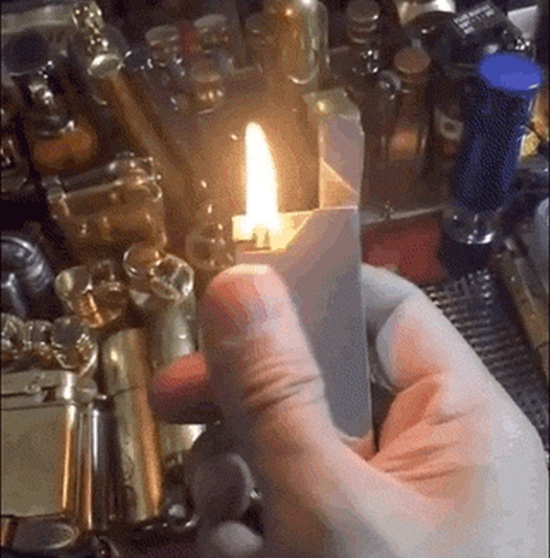A right hand, dusted from sanding, holds an upright lighter with the flame lit and the lid flipped open. The thumb is positioned on the front of the lighter, keeping it steady. The lighter sits above a silver mat, suggesting it could be a surface in a bar or a garage. Surrounding the lighter are approximately 20 metal canisters in the background, predominantly silver with a few blue and brass ones interspersed. The setting appears to be a workbench laden with various cylindrical and square objects, indicating a workspace filled with tools and materials.